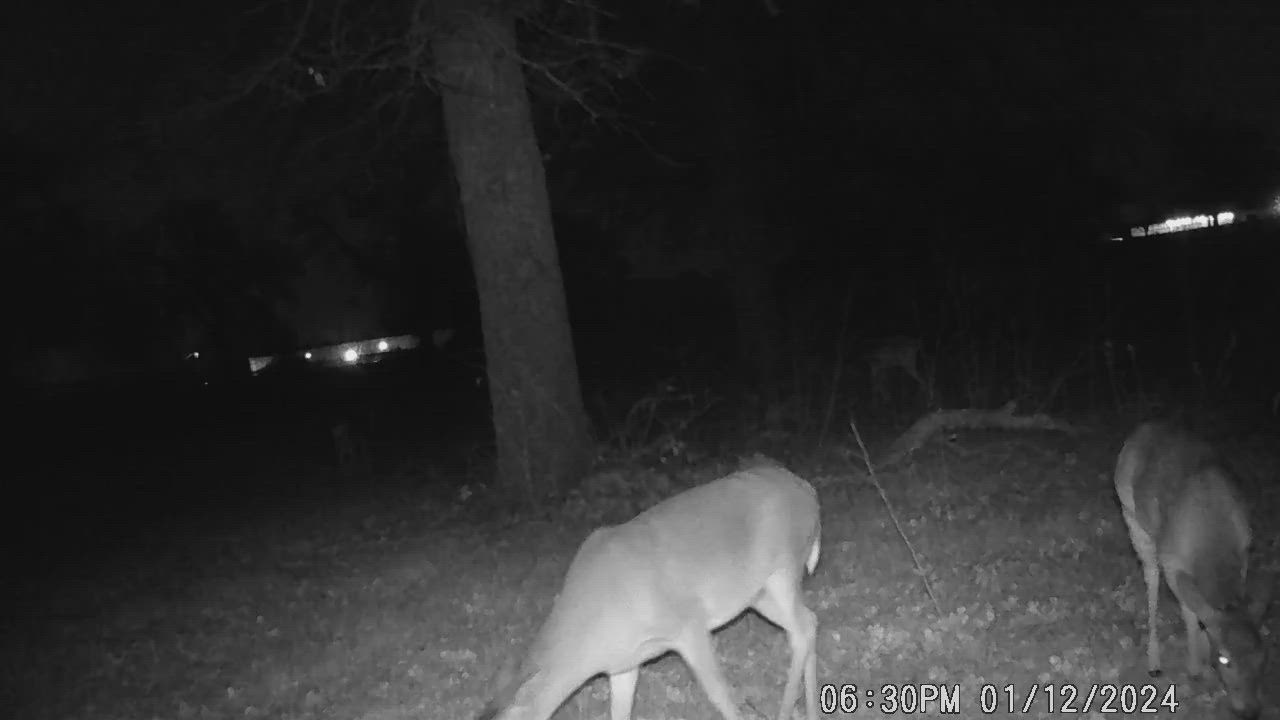This black and white photograph, taken by a trail cam at 6:30 PM on January 12, 2024, captures a serene nighttime woodland scene. The image, wider than it is tall, shows three deer grazing in a shadowy, wooded area. Two of the deer are prominently positioned in the foreground: one on the left with its head down, revealing its white tail, and the other at the bottom right corner, also with its head down, facing the camera. A third deer is faintly visible, further adding to the tranquility of the scene. There is a single noticeable tree slightly left of the center. In the background, faint residential lights suggest nearby houses, their porch lights subtly illuminating the scene.